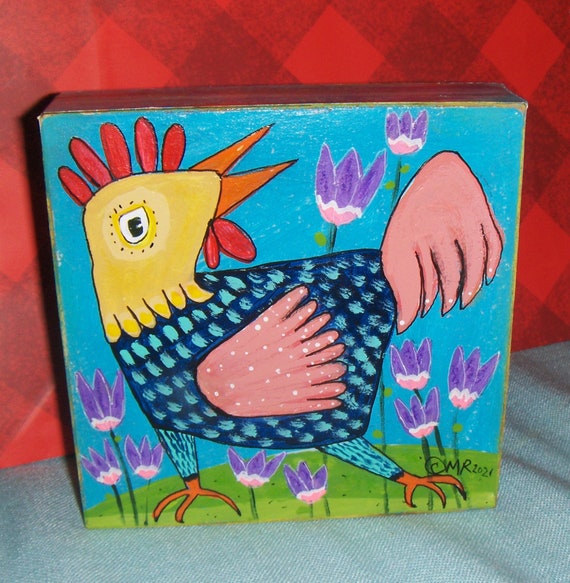This photograph captures a vibrant, detailed drawing of a multi-colored chicken set against a blue background. The chicken, featuring a yellow head, an orange beak, and red feathers atop its head, exhibits light and dark blue feathers on its body. Its wings are pink with white spots, while its orange feet and similarly pink tail add to its colorful appearance. Surrounding the chicken are clusters of purple flowers with white squiggles and pink bottoms, arranged with three flowers at the bottom left, two at the bottom center, three at the bottom right, and two at the top. The artwork is signed in the bottom right corner with "OMR 2024" in black writing. The drawing is framed within a square box that appears to sit on a pair of jeans, with a red checkered wall featuring X's in the background.